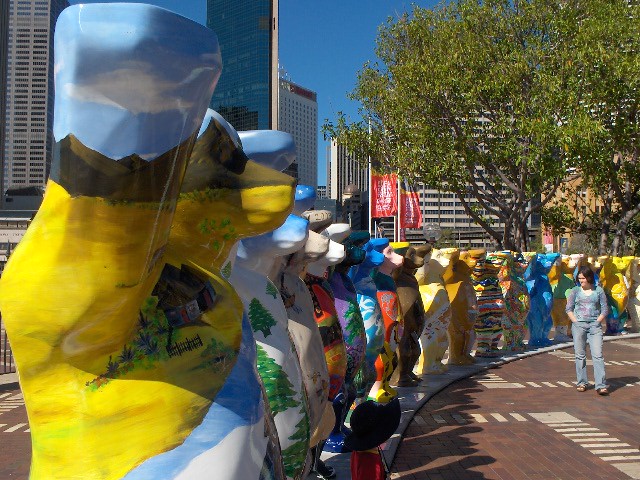The image captures a vibrant urban scene featuring a woman in faded blue jeans, a long-sleeved top, and sandals, standing on a curved pathway of brick pavers, closely observing a colorful exhibit of bear sculptures. There is also someone seated nearby, wearing a large sun hat. The bear statues, each about six feet tall and standing like humans with their right arms raised, are arranged side by side in an arc, forming the outer edge of what appears to be a circular park. Each bear is uniquely painted in bright colors, adorned with images of nature such as cottages, pine trees, and wooden fences, reflecting a variety of artistic styles. The setting is illuminated by a bright sunny day, with a large leafy tree and a backdrop of towering skyscrapers, suggesting it's amidst a bustling city.